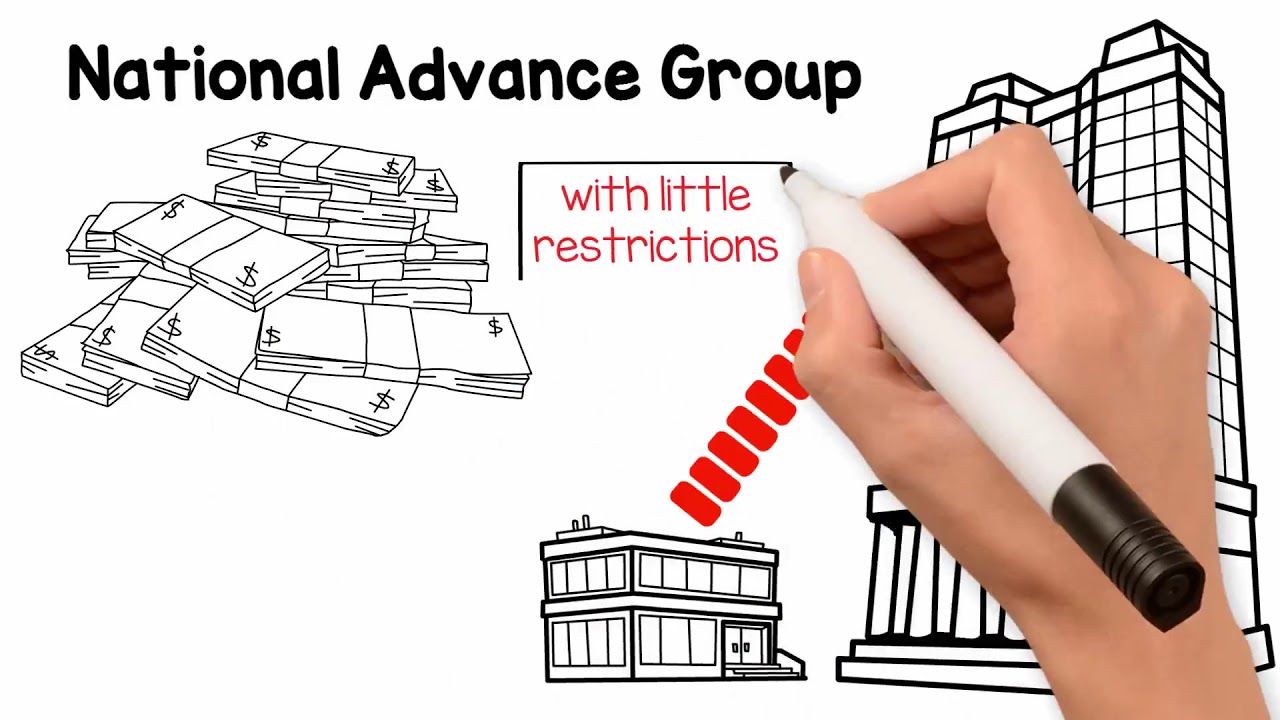The image depicts a detailed, black-and-white line drawing resembling a whiteboard sketch. In the upper left corner, the title "National Advance Group" is prominently displayed. Below the title, there is a neatly outlined bundle of stacked paper money. To the right of the money, a disembodied human hand, holding a white marker with a black tip and cap, is actively drawing. The hand is positioned on the right side of the image, outlining a half-rectangle around the words "with little restrictions," written in red. Below this text, towards the bottom, a small two-story building filled with windows sits centrally. To the right, slightly below the hand, a larger, tall building with numerous windows and large front columns stands prominently. The background is entirely white, emphasizing the hand-drawn elements.